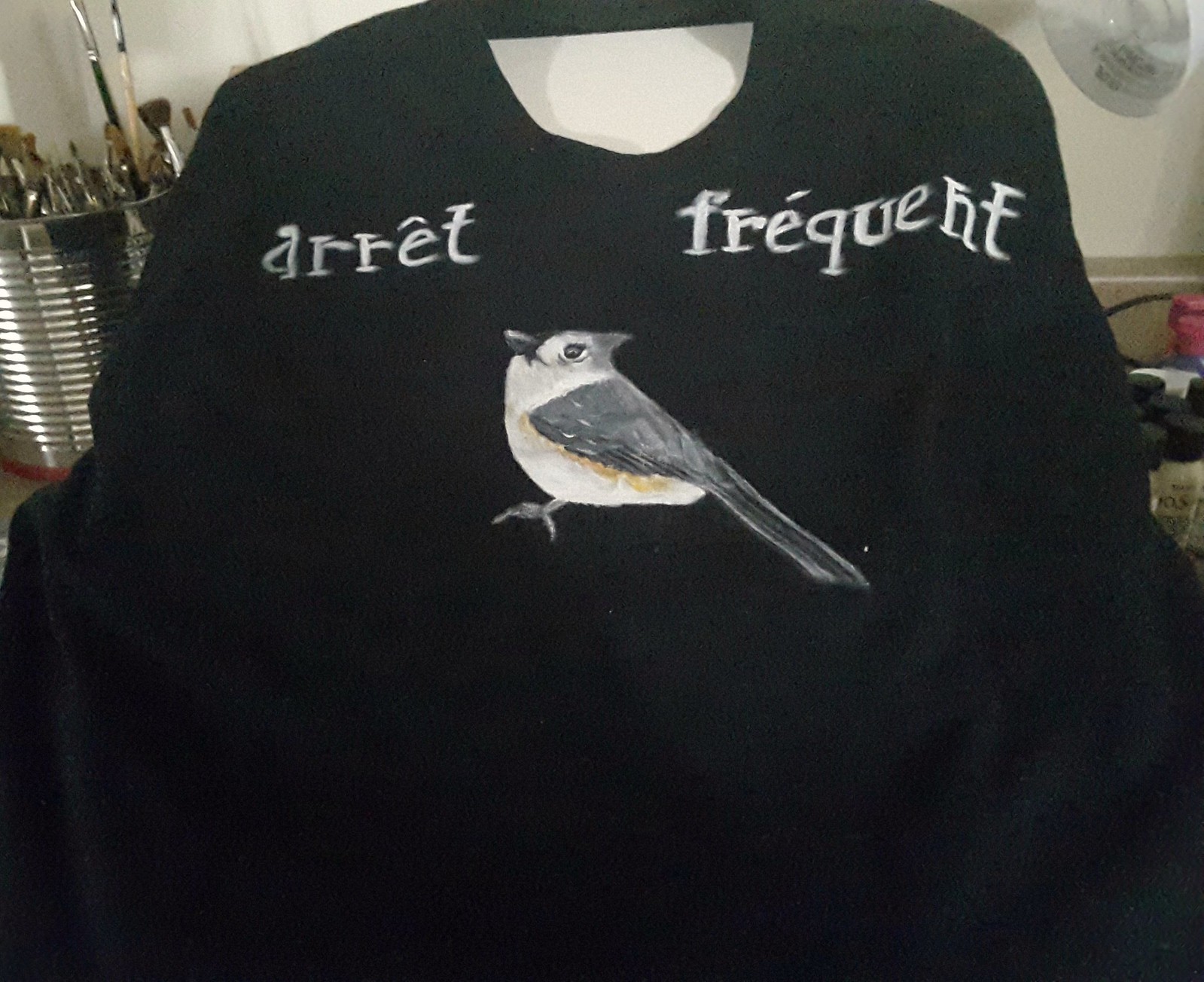This square photograph appears to capture a scene from an art studio. The foreground features an article of black clothing, possibly a sweater or apron, displayed upright. The garment has a cutout for the head and prominently displays a hand-painted design at the chest. The design includes the lowercase letters "a-r-r-e-t-f-r-e-q-u-e-n-t" with a small, gray and white bird resembling a cardinal, shown in profile facing left, just below them.

To the left of the garment, a silver metal container with horizontal ridges holds a variety of paintbrushes, their bristle ends pointing upward. On the right side, several small bottles with black caps are visible, inferred to be bottles of paint. Additionally, a mix of red caps are also visible among them. The background features a white wall, adding to the impression of a workspace. In the upper right corner of the image, a dangling white lamp can be seen, although it is not illuminated, suggesting natural light is being used. A white piece of cardboard is positioned behind the neckline of the garment, aiding in its display. The overall scene hints at a creative environment, possibly a kitchen repurposed as a painting studio.